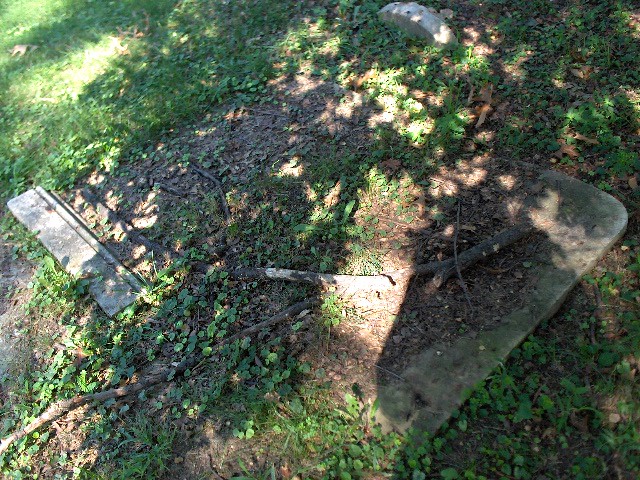In this outdoor photograph taken on a sunny day, the scene captures a plot of land characterized by dirt, grass, and various weeds. The area appears somewhat neglected, with a mix of green growth transitioning into more overgrown weeds and ivy. Scattered across the plot are what seem to be two flattened headstones, potentially indicating a cemetery, although it could also be an overgrown backyard with buried structures. There is a discernible shadow of a tree cast over the ground, though the tree itself is not visible in the frame. Additionally, the image shows several branches strewn about, with two larger branches and a few smaller ones lying across the stones. In the middle right of the photo, a rectangular fragment of stone partially protrudes from the ground, possibly the base of another headstone. Amidst the debris and dirt, the scene gives a sense of dilapidation and abandonment, punctuated by subtle details like the buried tip of a headstone barely visible at the top of the image.